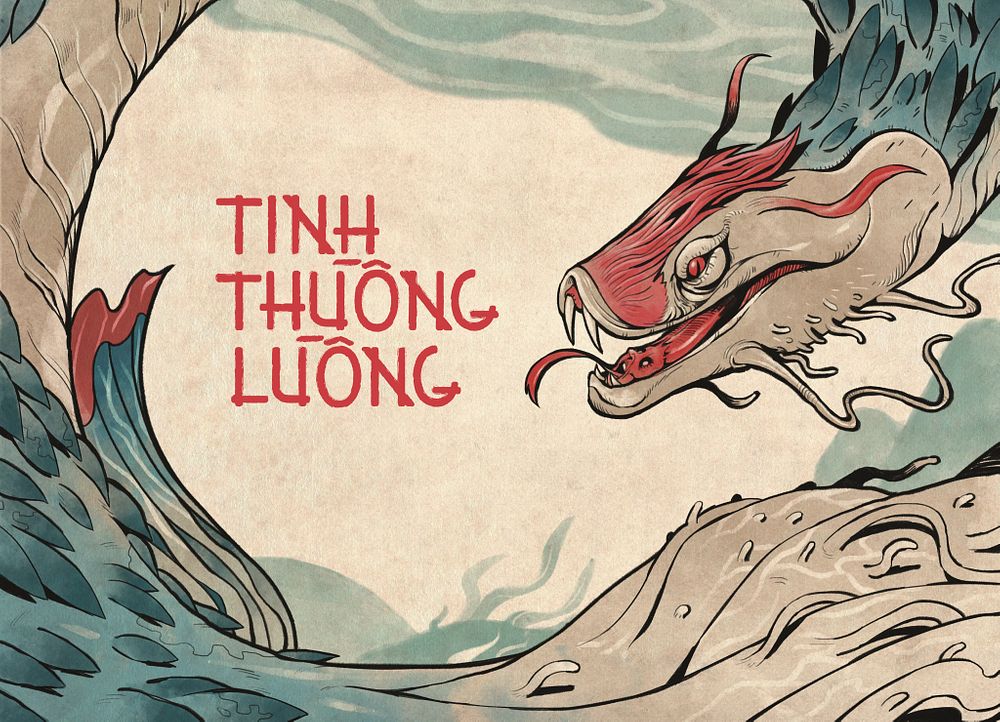The artwork portrays an Asian-style dragon with a serpentine neck and head resembling a snake. The dragon has a vibrant red tongue extending from its open mouth, which reveals two sharp fangs. There are small, tentacle-like appendages near its chin. The dragon's head, positioned to the right and facing left, seems to be gazing at the red text positioned centrally toward the left. This text consists of three lines in an Asian language, reading "T-I-N-H," "T-H-U-O-N-G," and "L-U-O-N-G," with diacritical marks above each "O" and "U." The dragon's partially visible body wraps around the left and bottom edges of the image, contributing to an encircling effect. The background is a tan-gray hue, reminiscent of a muted sky. Splashes of vibrant red on the dragon complement the red text, adding a striking contrast to the overall composition.